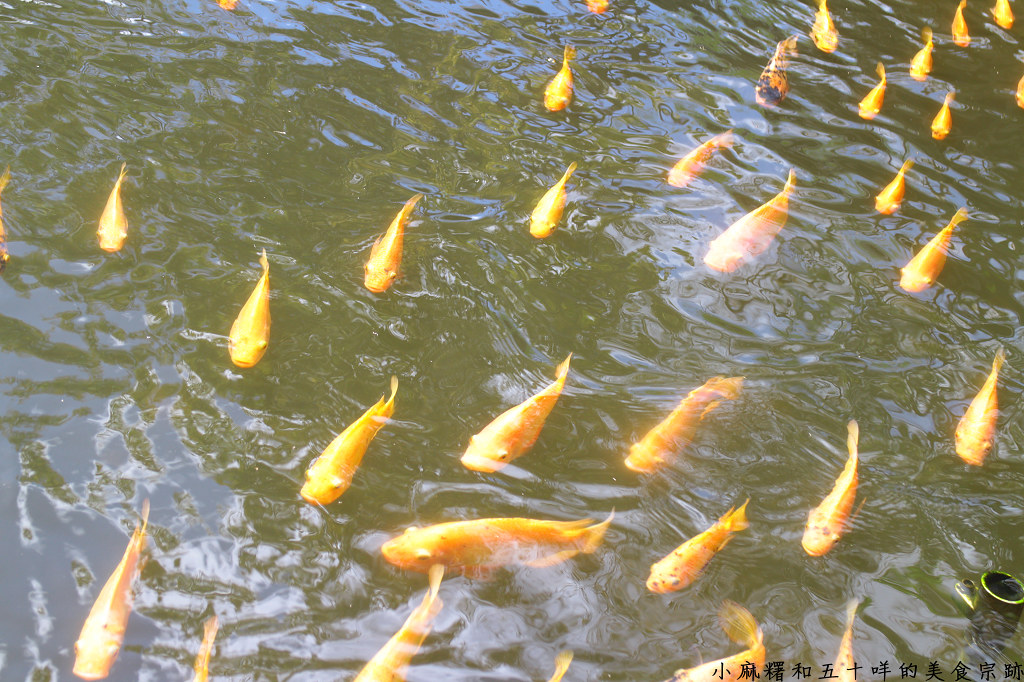This image captures a serene scene of numerous goldfish swimming in clear, rippling water. Most of the goldfish, with their sleek, elongated bodies, large eyes, and fanned tails, are brilliantly golden, though one distinctive fish features gold and black coloring. The fish are primarily moving from the top of the photo toward the bottom left, while one swims from right to left. The water is still, with slight ripples throughout, creating a peaceful ambiance. At the bottom right corner of the image, there's text in an Asian script, and a small shoreline with a golden ring adds an intriguing element to the scene. The setting appears to be an outdoor body of water, possibly a pond or canal, creating a natural and tranquil backdrop for the vibrant fish.